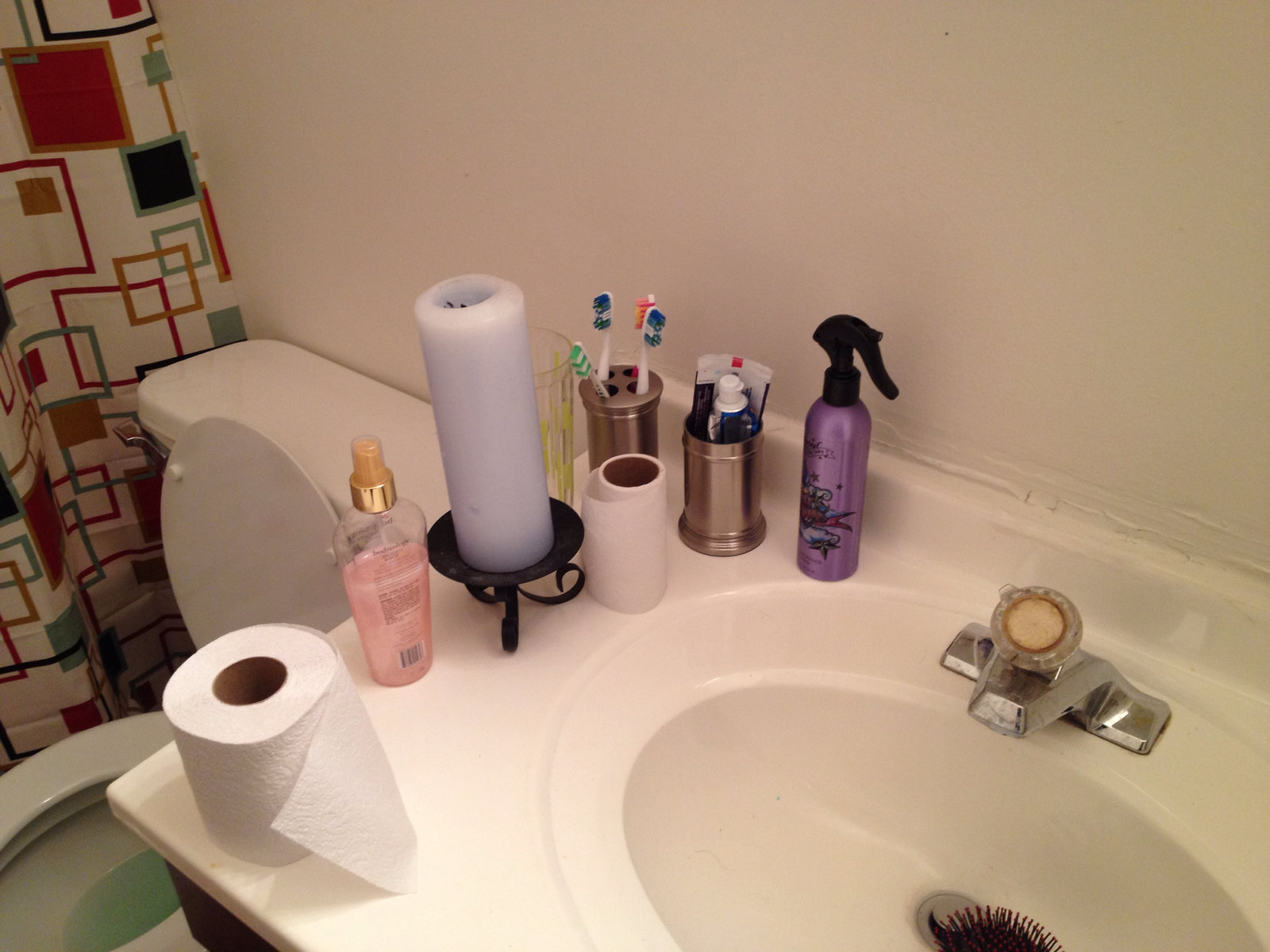This detailed photograph captures the intimate setting of a bathroom with predominantly white fixtures and various colorful details. The white porcelain toilet seat is up, revealing blue-tinted water inside, suggesting the recent use of a cleaner. Adjacent to the toilet is a shower curtain positioned on the left-hand side, characterized by a geometric pattern of squares in various colors, including pink, brown, dark blue, light blue, red, orange, olive green, purple, and light orange.

Moving to the sink area, which is an integrated unit with a white countertop, there's a cluttered yet organized array of items. Inside the sink lies a hairbrush with black bristles and pink tips. The sink features a silver stopper and a silver faucet with beige and gold accents bordered by brown. On the countertop are two rolls of toilet paper, one nearly depleted.

Among the items on the sink, there's a clear bottle of pink liquid with black writing and a golden lid equipped with a tan sprayer, likely a body spray. A gray candle sits on an ornate black saucer with curly Q legs, adding a touch of elegance. A drinking glass adorned with yellow flowers is partly hidden behind a toothbrush holder made of brass or metallic material. This holder organizes four different toothbrushes with varying bristle colors: green and white, blue and white, red, pink, orange, and a mix of dark blue, lighter blue, white, and green. Adjacent to the toothbrushes is another metallic holder containing multiple tubes of toothpaste. Completing the arrangement is a purple spray bottle with a black nozzle, perhaps a hair or room deodorizer.

Overall, the white walls and fixtures provide a stark contrast to the colorful details and various personal items arranged on the sink, creating a vivid snapshot of daily life in a household bathroom.